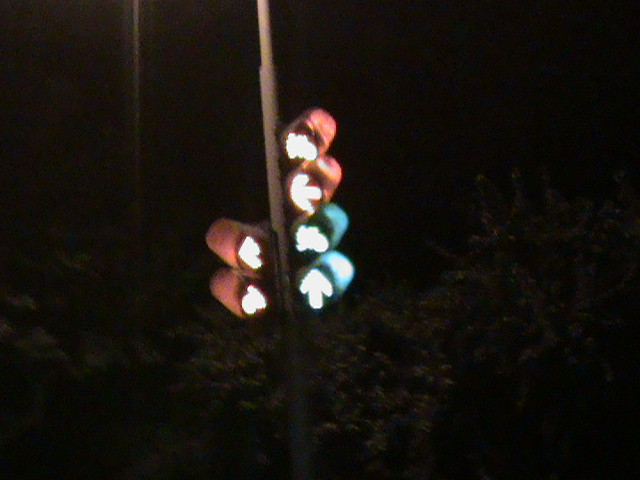In a photograph taken at night, a starkly black background frames a blurry yet intriguing scene featuring a row of illuminated traffic lights mounted on a pole. The image is dark and obscure, with vague shapes hinting at trees or bushes in the background. The lights themselves are more distinct, despite the overall poor quality of the photo. There are six circular lights, each encased in either a red or blue cover. 

On the left side of the pole, there are two traffic lights, both in red cases, displaying an arrow pointing to the left and a symbol resembling a bicycle. On the right side, there are four more lights: the upper two have red cases showing another left arrow and an up arrow, while the lower two, in blue cases, depict similar symbols. All lights emit a consistent white glow, creating a striking contrast against the darkness and drawing the viewer’s gaze. Despite the blurred image, the arrangement and vividness of these lights offer a glimpse into an array of directional and symbolic signals.